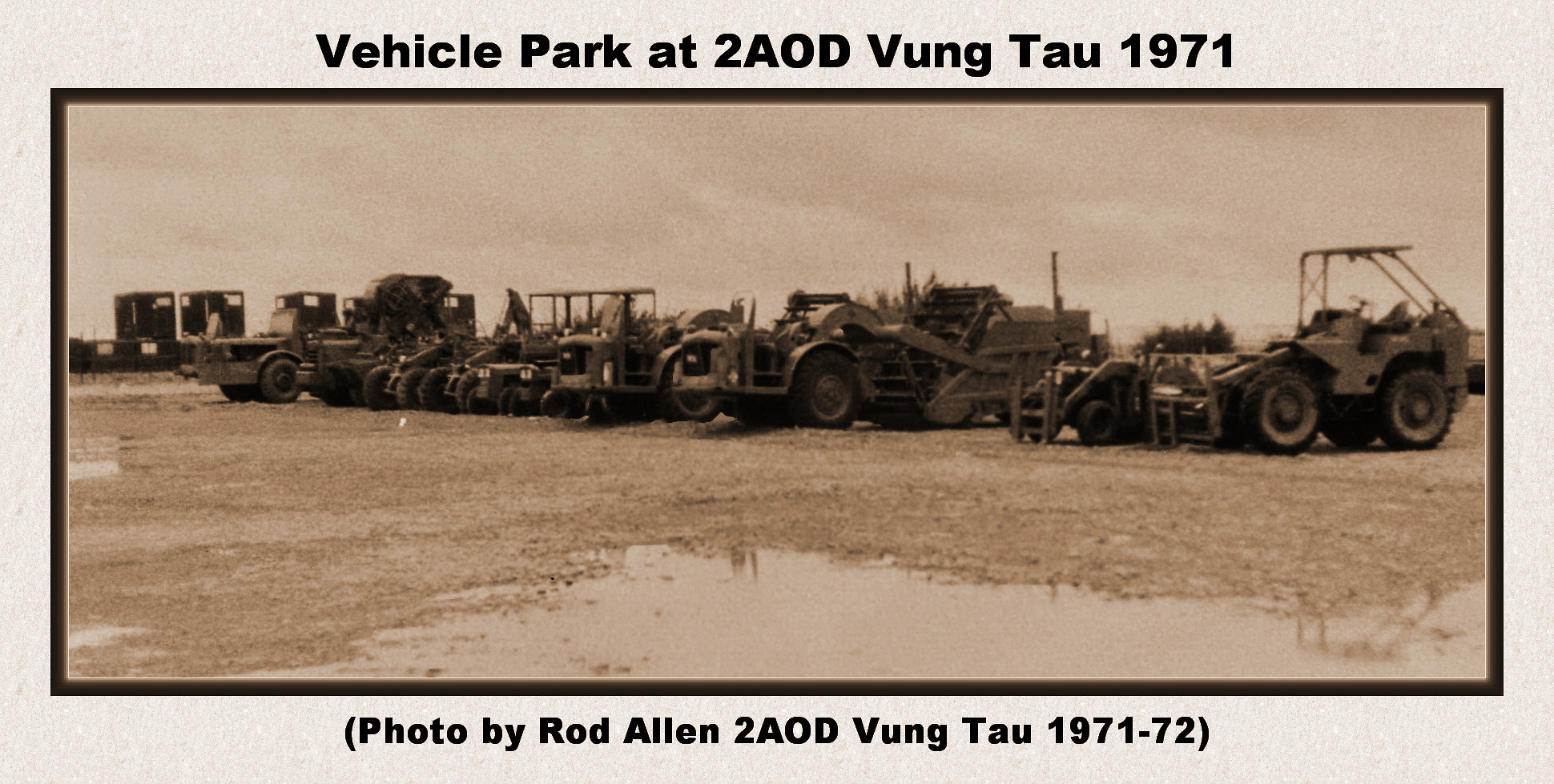This image captures an old, brown-tinted photograph from 1971, set in Vung Tau during the Vietnam War. Encased in a light tan border with a darker brown strip outlining the photograph itself, the image bears the title "Vehicle Park at 2AOD Vung Tau 1971" at the top, and credits "Photo by Rod Allen, 2AOD Vung Tau, 1971-1972" at the bottom. The photograph, oriented horizontally, displays a wide-angle view of various military vehicles—likely construction equipment such as earth movers—arranged in the center of a muddy, barren field. Dominating the lower part of the image, a large puddle anchors the foreground, with additional puddles visible to the left. The vehicles, totaling around eight, have large tires and open tops, hinting at their use in heavy-duty construction or farming activities. The overall setting appears overcast and the photograph's brown tinge adds a nostalgic, sepia effect, emphasizing the rugged, outdoor conditions of the time.